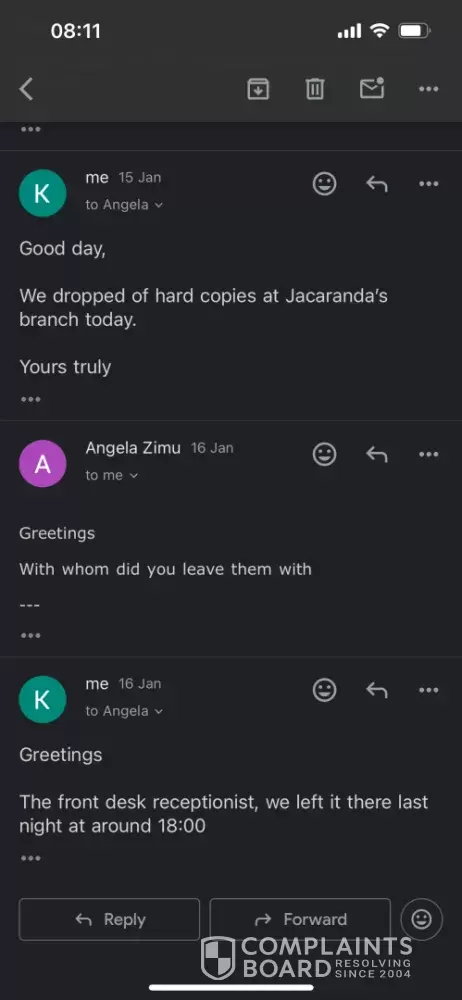A screenshot captures an iPhone screen at exactly 8:11 AM, evidenced by the time displayed at the top left corner. The device shows full network signal strength, as indicated by the bars at the top right. Adjacent to the network signal, the Wi-Fi icon is visible, confirming a strong connection, and the battery icon displays a high charge level, indicating that the device is sufficiently powered.

The open application appears to be the Gmail app, displaying an email conversation. The initial message is titled "Good day," in which the sender, Angela Zemo, informs the recipient that hard copies were dropped off at Jacaranda's branch the previous day. In subsequent lines of the conversation, Angela inquires about the exact person with whom the documents were left. The recipient of the email responds that the hard copies were handed over to the front desk receptionist the previous night at approximately 6 PM. This detailed exchange between Angela Zemo and the recipient highlights essential information about the document submission process.